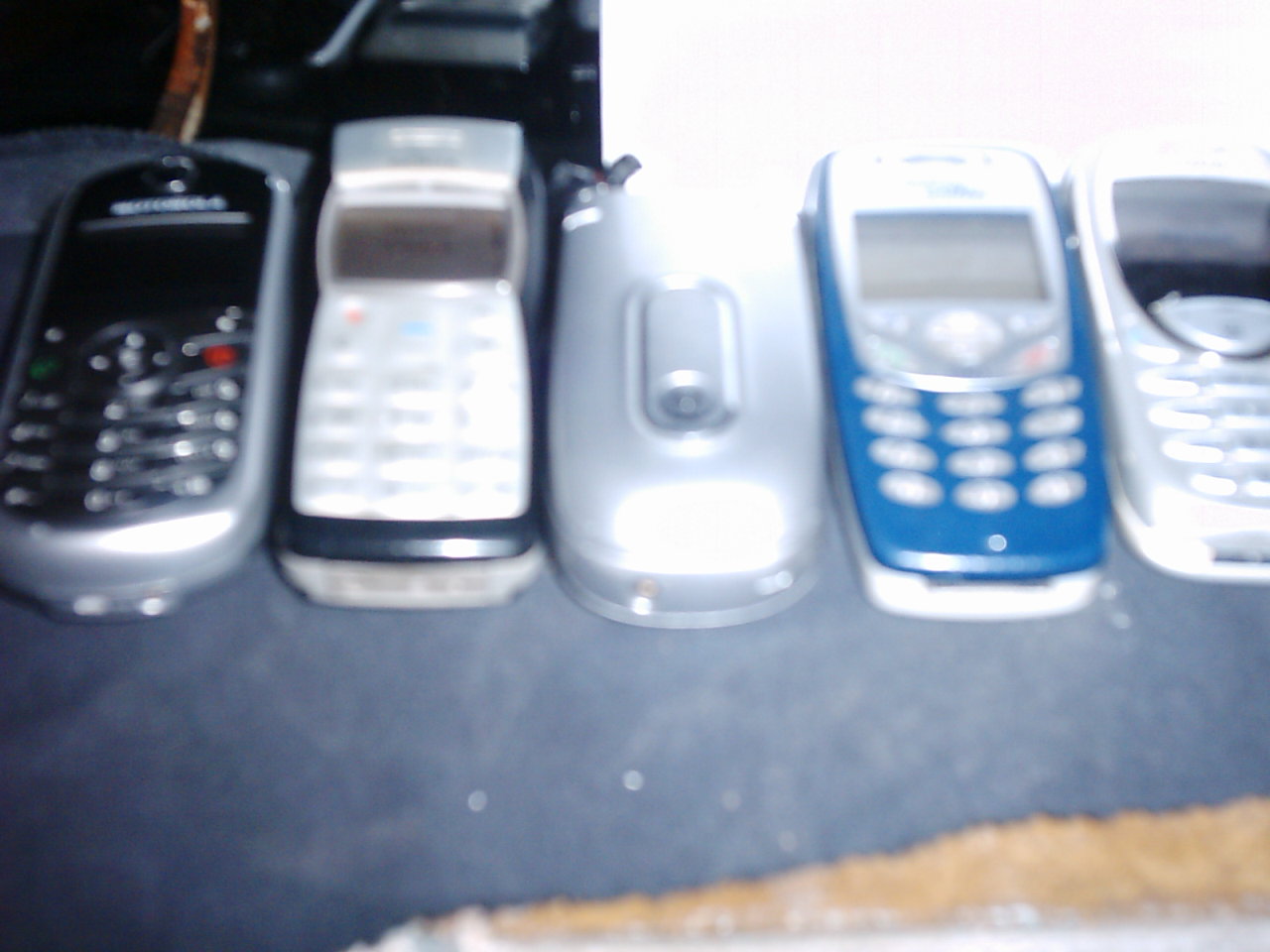This is an image depicting a row of five old cell phones arranged on a gray table. Each phone hails from the early era of mobile technology, characterized by physical keypads rather than touch screens. 

Starting from the left, the first phone features a silver body with a black keypad and display area. The second phone, silver with a black outline around a small black screen, also has more noticeable details. At the center is a closed silver flip phone, distinctly different from the others, which all have visible keypads. The fourth phone stands out with its blue lower section and silver buttons. Finally, the fifth phone is silver with silver buttons and a small black screen, slightly blending into a potential light silver lower section. 

The backdrop includes a gray table with hints of a brown paper or cloth at the bottom right and a black surface beneath the phones. The overall image is slightly blurry, making finer details somewhat difficult to discern. The setting likely aimed to showcase the collection, possibly for nostalgia or resale purposes.